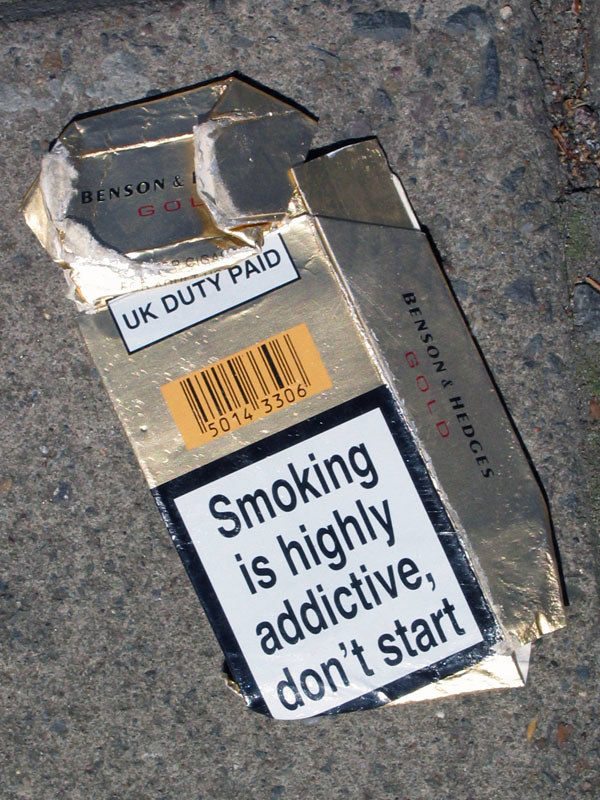The rectangular photograph, approximately six inches tall by four inches wide, captures a ground-level view of grayish-blue cement pavement, speckled with small rocks. In the upper right-hand corner, the pavement is chipped and littered with bits of dead leaves. Dominating the image is a crumpled silver cigarette pack, likely metallic gold in its original state, starting from the lower right and extending towards the upper left corner. The pack is significantly flattened and bears signs of use. Prominent on the back is a white square with a black border that reads, "Smoking is highly addictive, don't start" in bold black letters. Above this warning is an orange box containing a barcode. Towards the upper part of the package, a white rectangle outlined in black states "UK Duty Paid" in capital letters. The side of the pack features the text "Benson & Hedges" in black vertical print, with "Gold" written underneath in red. The top of the pack, crumpled and folded in, also displays the text "Benson & Hedges Gold." The image distinctly shows the intricate details of the damaged cigarette packaging against the rough texture of the pavement.